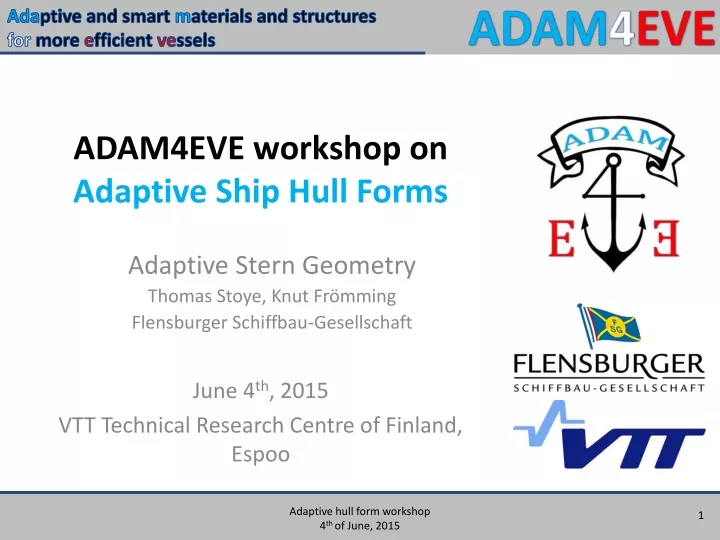This image appears to be part of a larger presentation, indicated by the “1” in the lower right corner. The slide has two beige horizontal borders at the top and bottom. The top border features the text “Adaptive and smart materials and structures for more efficient vessels” on the left and “Adam for Eve” on the right, with Adam in blue, 'for' in white, and Eve in red. The center of the slide showcases a workshop invitation in various fonts and colors. At the top, in black text, it reads “Adam for Eve Workshop on”, followed by “adaptive ship hull forms” in blue text, and “adaptive stern geometry” in gray text. Below this, it lists the presenters, "Thomas Doyle, Nutt Fromming," and includes the date “June 4th 2015”. The bottom beige border reiterates the event details in small black text: “Adaptive hull form workshop, 4th of June 2015.” Several logos appear to the right, including a banner with 'Adam' in blue, an anchor, and both 'E's forming the word 'Eve', along with a blue VTT symbol. The background is predominantly white, and this slide appears to advertise a technical research workshop hosted by the VTT Technical Research Center of Finland.